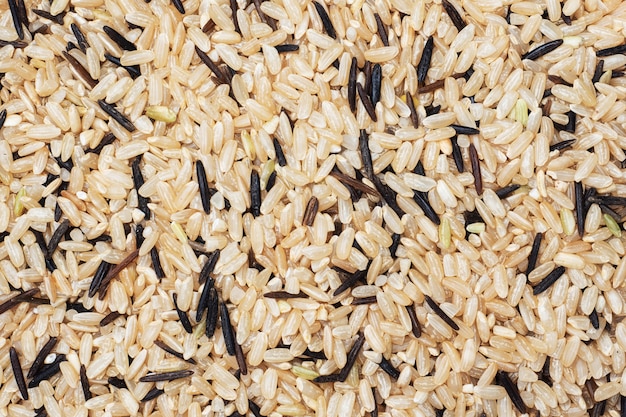The image captures an overhead view of a blend of uncooked rice grains spread out to fill the entire frame, which is a horizontal rectangle, approximately one and a half times wider than it is tall. Most of the rice grains are beige, typical of white rice, interspersed with longer, darker grains indicative of wild rice. These include brown and black grains, which add texture and color variation to the scene. A few grains even exhibit a slight green tint. The rice appears tight and not yet plump, suggesting that it has not been cooked. The overall aesthetic of the image showcases the contrasting colors and textures of the mixed rice varieties, with a clean and visually appealing appearance.